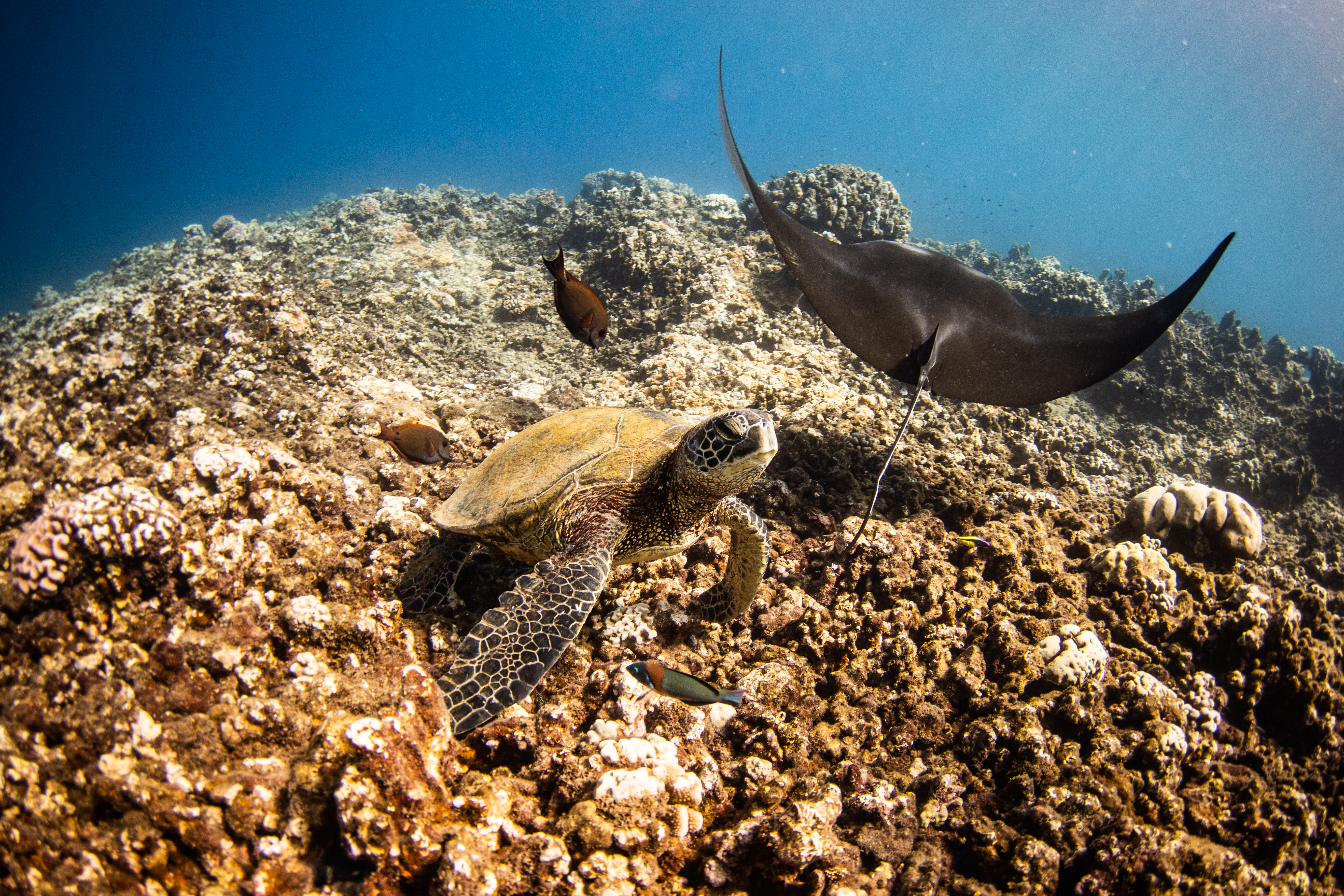In this captivating underwater image, the scene is bathed in a serene blue hue. The background water is an enchanting deep blue, illuminated by a gentle beam of light streaming from the upper right corner, casting a subtle glow over the entire image. In the foreground, a curious turtle with a yellowish-brown shell glides gracefully through the water. His leathery flippers are extended outward, showing no sign of fear, while his neck is stretched upward, and his eye is focused intently on the camera, creating a moment of serene connection.

Accompanying the turtle, a dark blackish-brown stingray elegantly cruises through the water. Its flat body and flippers arc upwards, giving it a sleek and streamlined appearance. The stingray’s long antenna-like appendages extend from its front, delicately brushing against the vibrant coral reef beneath.

Adding to this stunning aquatic tableau, two small fish make an appearance. One, positioned near the front, is a tiny black fish with hints of red, displaying an oblong shape. The other, swimming slightly above, is shaped like a horizontal teardrop with a visible little flipper at its back. Together, these elements create a mesmerizing snapshot of underwater life, full of detail and teeming with vibrant marine life.